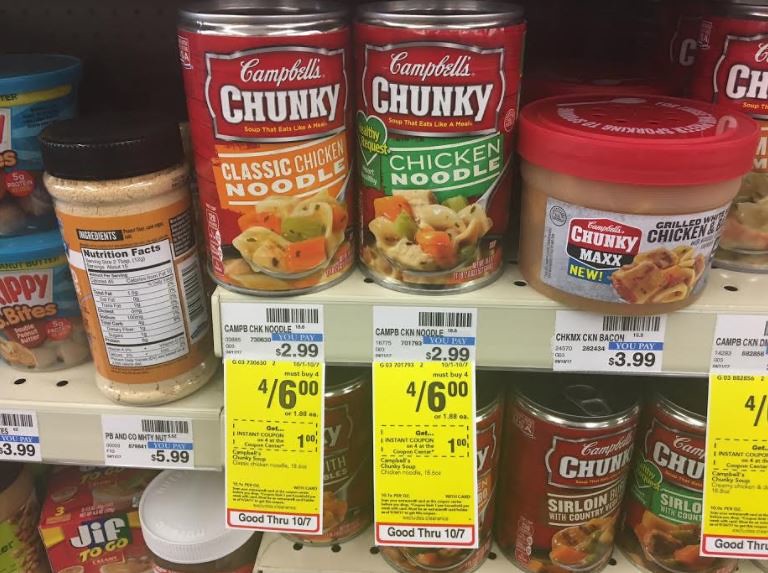This horizontally-oriented color photograph captures a supermarket aisle with four neatly arranged shelves filled with various grocery items. The top two shelves predominantly feature Campbell's Chunky Noodle Soup in a variety of flavors, stacked in rows creating a bright display of red, yellow, green, blue, and orange-labeled cans. To the bottom left-hand quarter of the image, there’s a display of peanut butter, with Jif jars occupying most of the space and Skippy peanut butter jars situated above them. The metal shelves, painted in a white-beige color and characterized by perforated holes, add an industrial aesthetic to the setting. Attached to the shelf edges are price tags, with notable sales highlighted; Campbell's Chunky Classic and Chicken Noodle soups are promoted at four cans for $6. The overall lighting is provided by overhead tungsten lights, imparting the photograph with a slightly warm, yellowish hue. The organized layout, vivid colors, and detailed product arrangement evoke a sense of variety and abundance typical of a well-stocked supermarket.